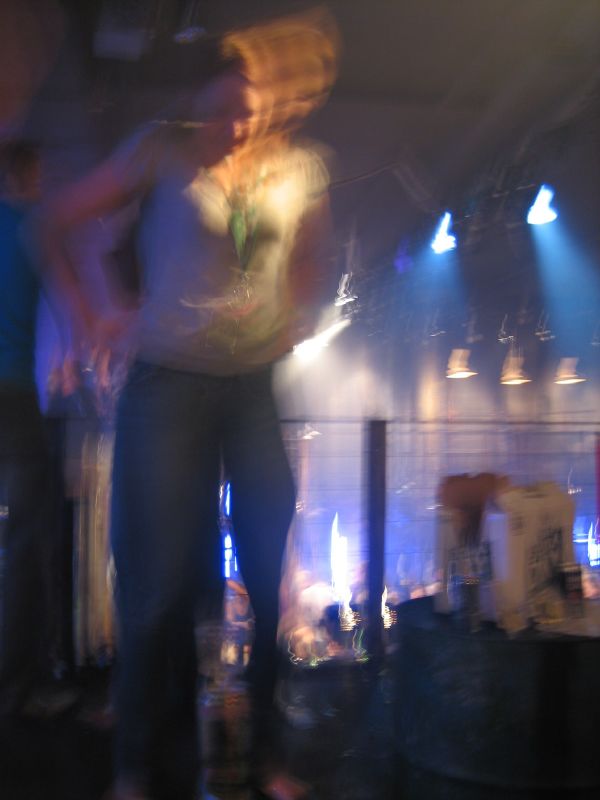In this extremely blurry photograph, the focal point is a woman with red hair, though some might perceive her as a brunette due to the photo's poor quality. She's wearing a white tank top and dark pants, possibly black or blue denim jeans, paired with boots. Around her neck, she sports a large round green necklace, standing out distinctly in the image. Her arms are pressing against her sides, contributing to the sense of motion that the blur captures. 

The setting appears to be a lively club or bar, characterized by a high ceiling adorned with multiple hanging pendant lights and other light sources creating a mix of blue hues. Behind her, the background reveals a band performing, and an area filled with other patrons either dancing or moving around, suggesting a bustling, energetic environment. Scattered on the floor are various objects, likely bottles, cans, and perhaps a box, contributing to the chaotic yet vibrant atmosphere of the scene.